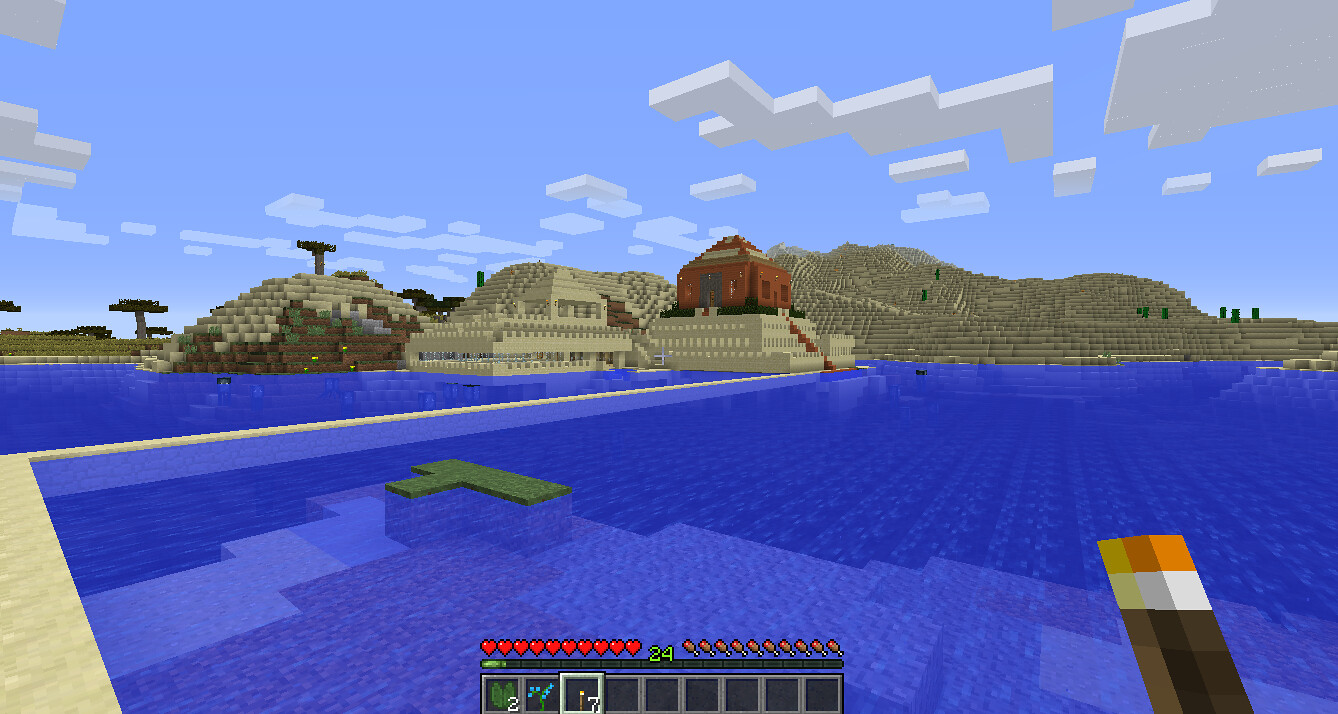A vibrant video game landscape is depicted under a bright blue sky, where whimsical, Lego-like clouds in various shapes—squares, C-shapes, and L-shapes—float overhead. Dominating the terrain are gray-topped hills armed with formidable cannons. The scene includes several light gray tanks poised for action and features both large hills and smaller rocky protrusions in the distance. A substantial body of water stretches out, punctuated by a concrete barrier and an L-shaped structure emerging from its depths. Adding to the eclectic mix, a tall, multicolored tower in shades of brown, white, and orange rises prominently, adding a dynamic element to this imaginative and detailed digital battleground.